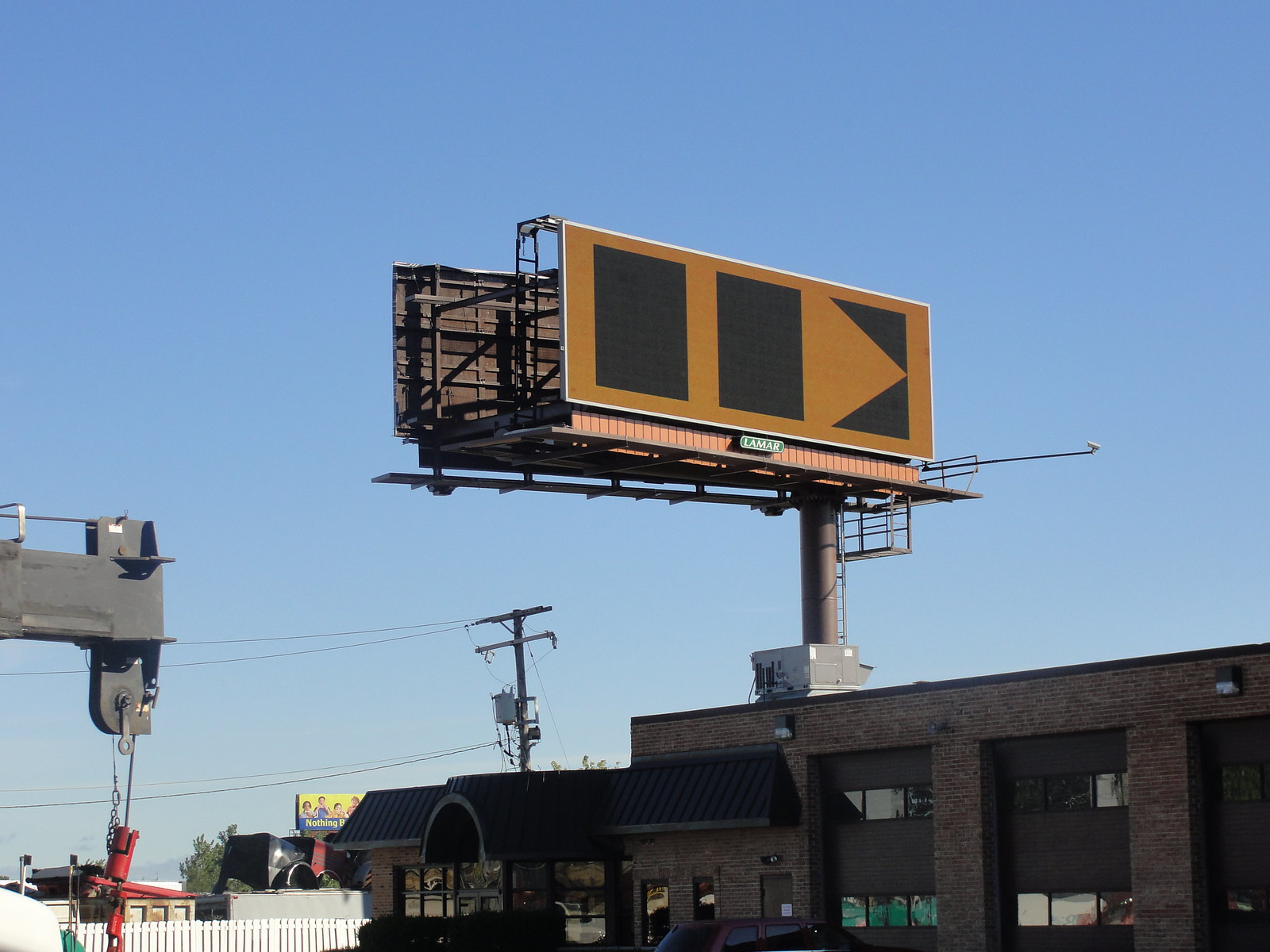This photograph features a prominent red brick building, characterized by three large doors indicative of a mechanic’s garage, alongside an office section adorned with black awnings over its windows and entrance. Atop the building stands a colossal billboard, supported by an intricate metal pole structure primarily on the right side. The billboard, resembling the size of a railroad car, flaunts a brown background with three distinct figures: two solid black triangles and a third figure that appears as a modified rectangle with a triangular cutout from its upper left side toward the center, reminiscent of a Pac-Man figure. The steel structure also includes dual platforms and lighting structures that cast light back onto the billboard. The detailed backdrop reveals another billboard, extensive sky, some phone lines, and various equipment, including a crane and a gray metal apparatus supporting a red object, emphasizing the bustling industrial ambiance. The visible logos, including Lamar and a green sign beneath the billboard, add to the complexity and functionality of this imposing advertisement structure, which appears to be under construction.